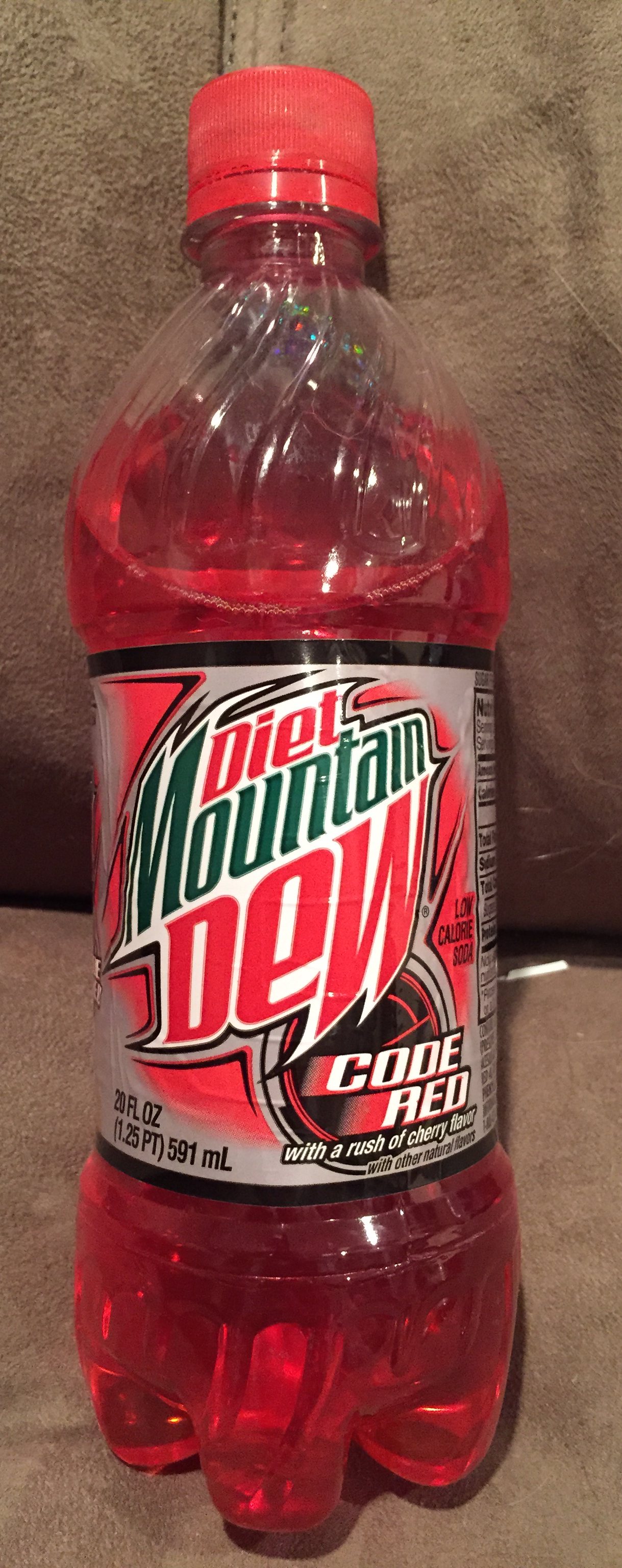The close-up image displays a nearly full 20-ounce plastic bottle of Diet Mountain Dew Code Red with a red cap, positioned on what appears to be a textured, brownish leather or suede chair or sofa. The clear bottle, containing a red liquid, is tilted slightly, indicating a small amount has been consumed. The label features a predominantly silver background with red and black accents. The branding includes "Diet" in red, "Mountain" in green, and "Dew" in red, with the "Code Red" insignia to the bottom right, accompanied by the text "with a rush of cherry flavor." The image's narrow, vertically rectangular frame highlights the textured, dark tan to light brown backdrop.